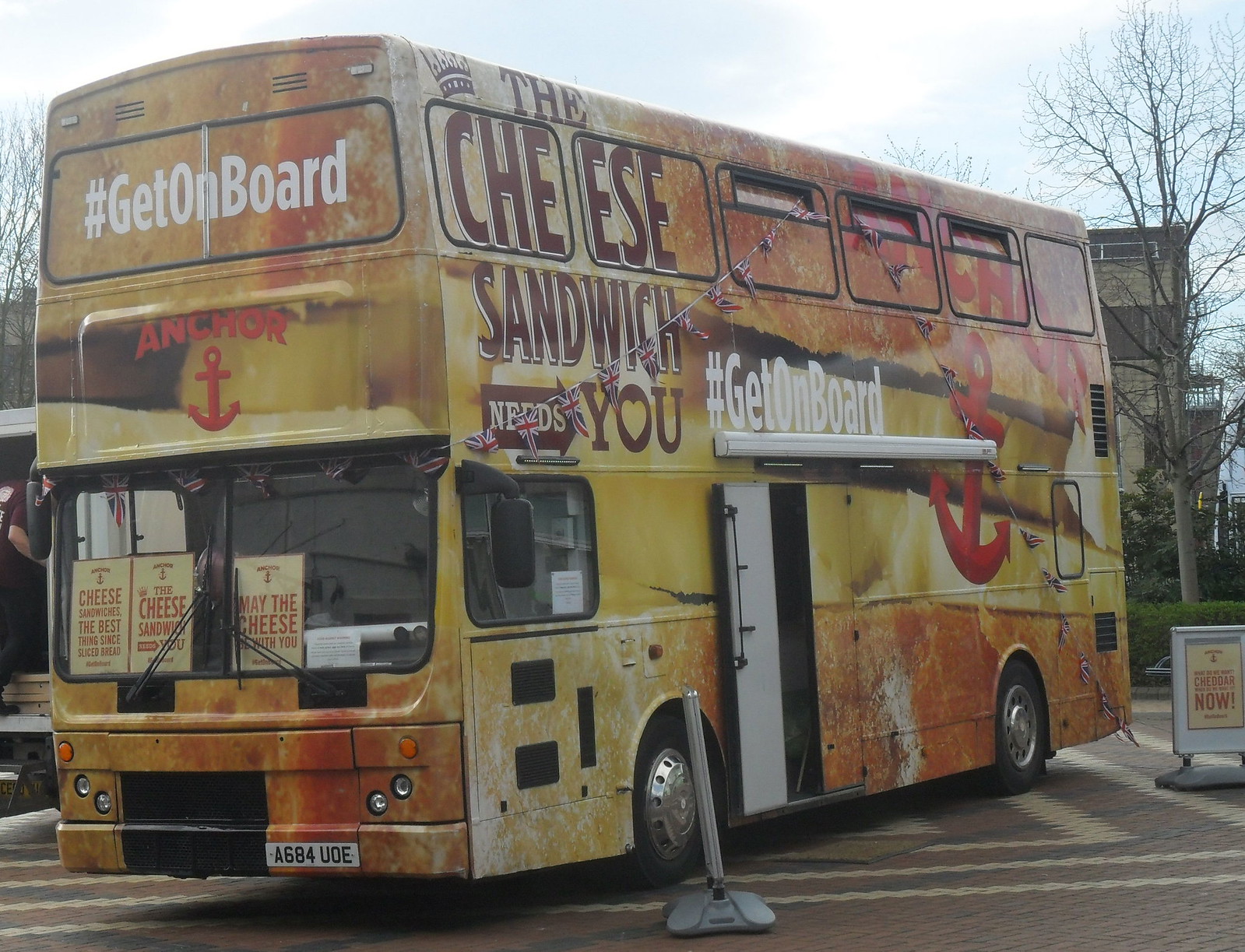The image depicts a double-decker bus retrofitted into a mobile restaurant that focuses primarily on cheese sandwiches. The front of the bus is adorned with the hashtag "#GetOnBoard" under a red anchor image. Through the bottom portion of the bus's windshield, partially legible text reads "cheese sandwich the best" followed by an illegible part. Additional signage on the bus includes slogans like "The cheese sandwich be with you" and "May the cheese be with you," emphasizing its cheese-themed menu. The middle section of the bus has an open door, indicating that the restaurant is operational. The bus, equipped with silver hubcaps and black wheels, is parked in an asphalt lot marked with white striping, next to a tree with no leaves and a nearby metal pole. The overall scene captures the bus as a stationary, yet mobile, establishment on a semi-sunny, cloudy day.